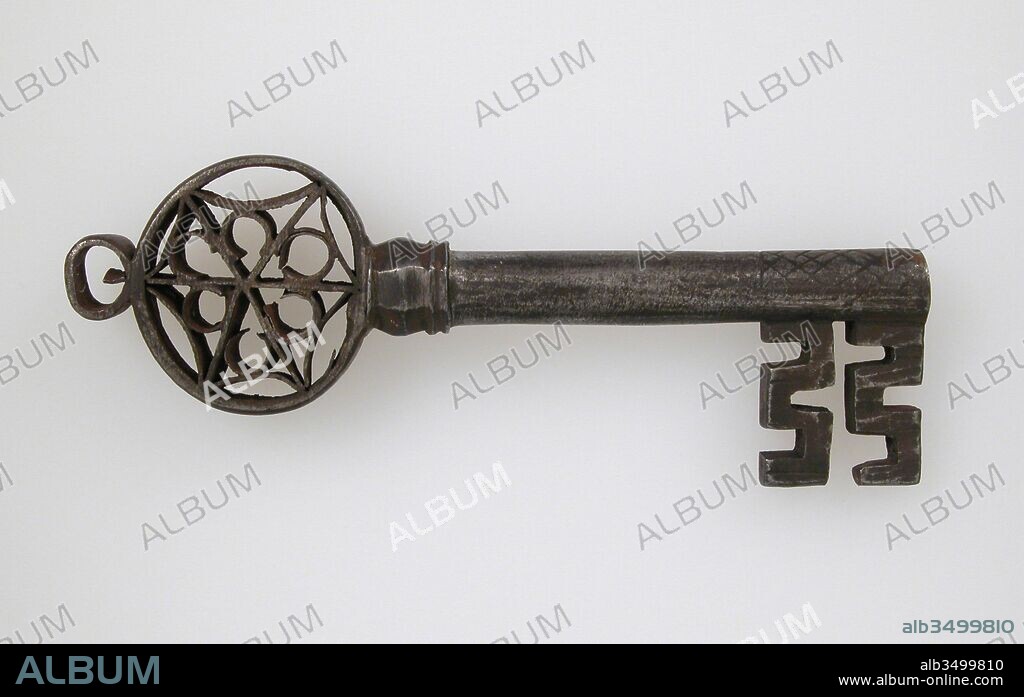This image is a horizontal, close-up photograph of an antique key with an ornate design. The handle, located on the left side, features a large decorative circle adorned with an intricate web and circle pattern. The key extends to the right in a straight, thin metal bar, ending in two identical zigzag shapes that represent the teeth of the key, designed to fit into a keyhole. The background is a very light gray with dark gray and white watermark text repeatedly saying "album" diagonally across it. Along the bottom of the image, there is a black bar with dark gray text on the left reading "album" and white text on the right displaying "ALB3499810" alongside the website "www.album-online.com." This image emphasizes the old-fashioned, detailed craftsmanship of the key against a subdued, text-branded background.